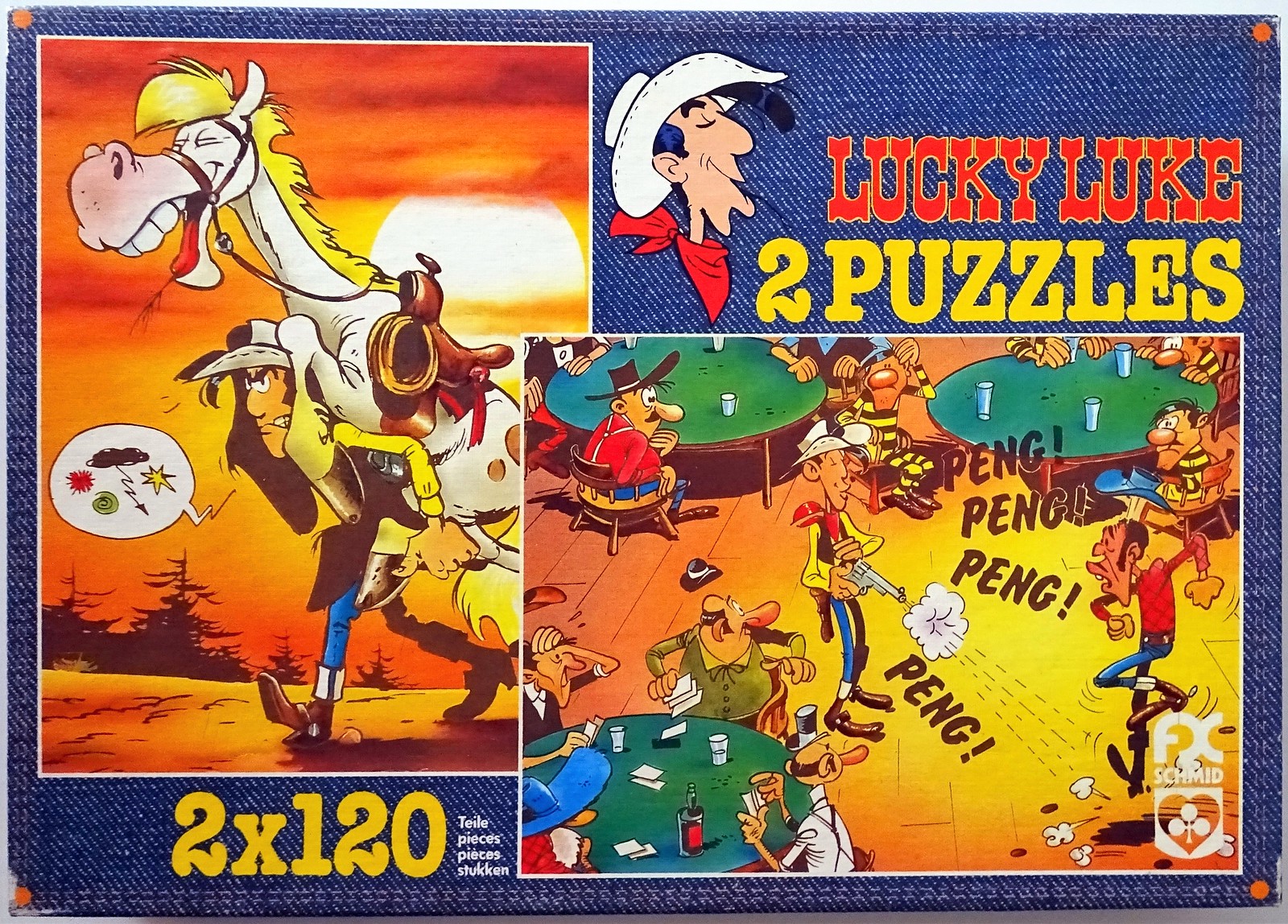The image is the cover art of a puzzle box featuring characters and scenes from the "Lucky Luke" series. The background resembles blue denim accented with red dots in each corner. Dominating the left side, there's a cartoonish illustration of a white horse with brown spots and a blonde mane, laughing with its mouth open, while being carried by an irate cowboy named Lucky Luke. Lucky Luke is depicted in typical western attire, including a white cowboy hat, a red handkerchief, a brown vest, blue pants, and brown shoes. Symbols indicating explicit speech (a red "POW" symbol, a yellow star, a black arrow from a cloud, and a green circle) emerge from his mouth, suggesting frustration.

On the right side, another cowboy is seen chewing on a tumbleweed and wearing a red bandana. Text next to him in orange and yellow letters reads "Lucky Luke" and "Two Puzzles," respectively. Below this, another scene shows a cowboy in a white hat shooting a pistol with comic "PING PING PING" sound effects. He’s disrupting a bar scene where multiple characters, including some dressed in black and yellow striped jail outfits, are engaged in drinking and playing poker.

Text throughout the image indicates "2x120" and "120 Pieces" suggesting two 120-piece puzzles are included in the box. The colorful and lively illustrations capture the humorous and adventurous spirit of the Lucky Luke series.